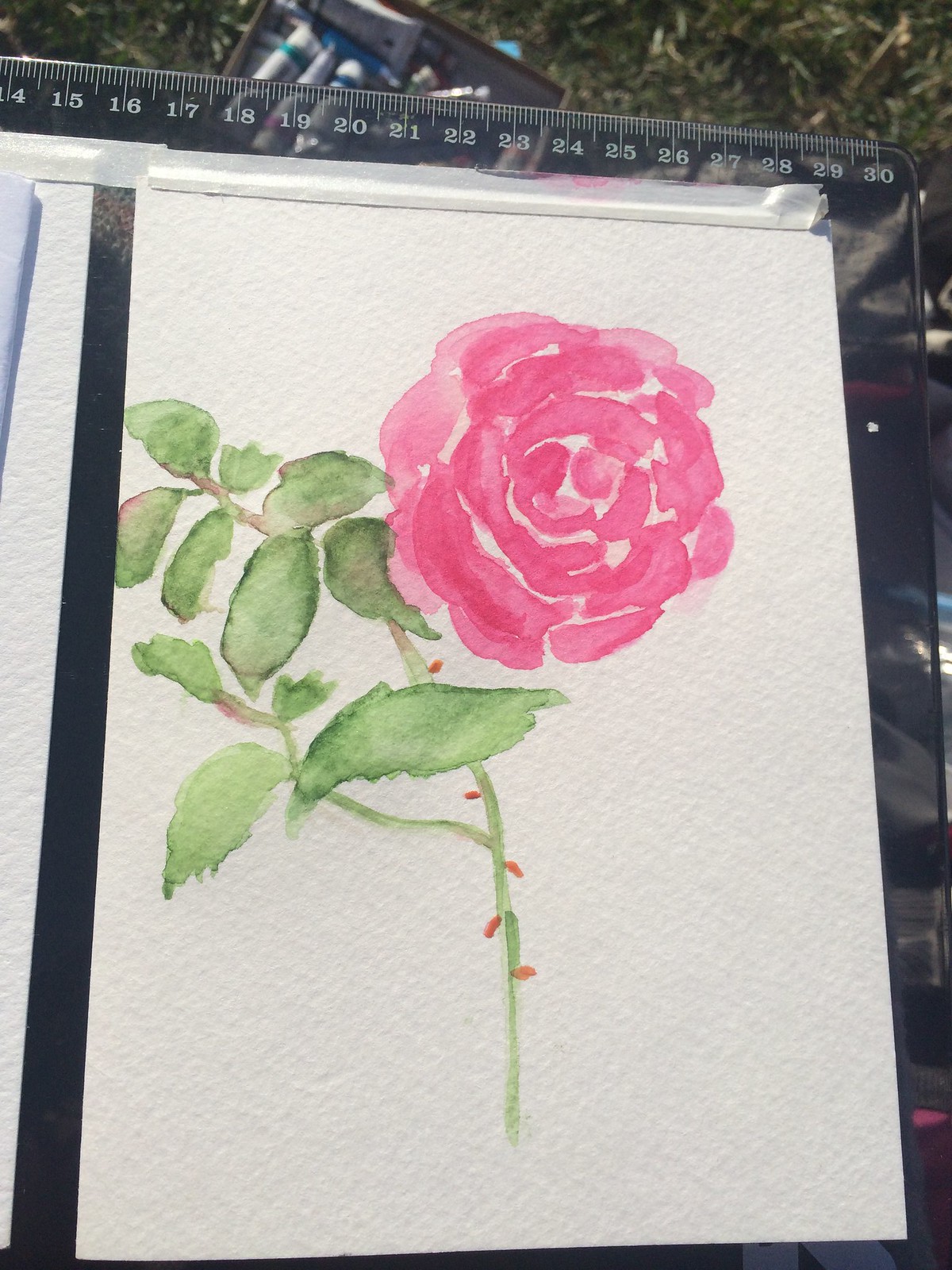This captivating watercolor painting, rendered on subtly textured white watercolor paper, is meticulously measured from 16.5 inches to 29 inches in width, as indicated by the ruler placed beneath it. The composition showcases an exquisite pink rose, meticulously depicted with intricate detail. The rose features a central cluster of three delicate blotches, surrounded by three sequences of petals which progressively expand outward, creating a mesmerizing floral bloom in various shades of medium pink.

The slender, graceful stem of the rose is painted in a thin green hue, delicately adorned with what appear to be small, pale orange thorns that lack pronounced sharpness. A secondary stem extends from the main one, maintaining the organic composition. Complementing the scene are a few light green leaves, adding an extra layer of natural beauty. The right side of the painting is slightly obscured by a small strip of plastic, leaving a trace of mystery about the painting's surroundings, possibly suggesting an outdoor setting. This watercolor artwork captures the intricate simplicity and natural elegance of a single rose in full bloom.